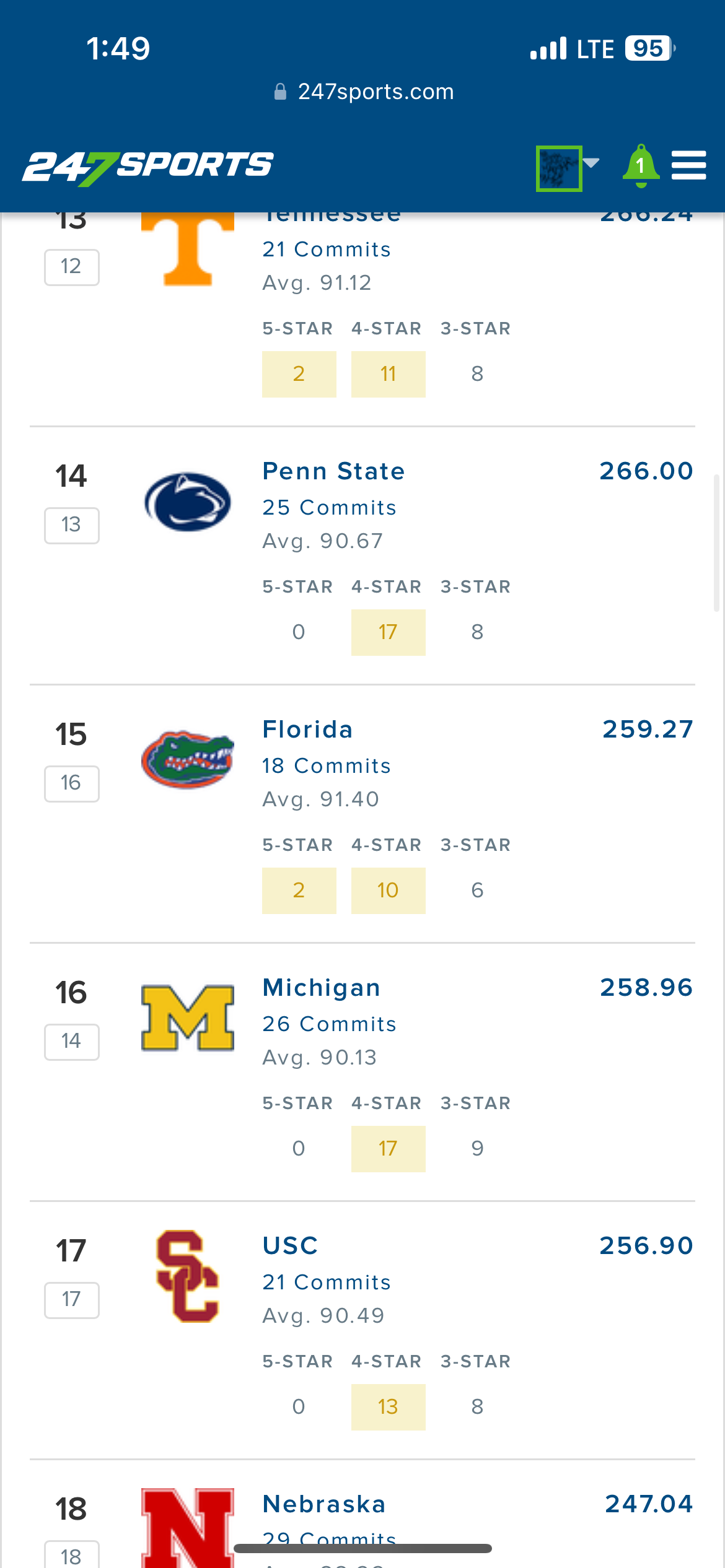This image features the interface of the 247Sports mobile application displayed on a smartphone. At the very top center of the screen, the header reads "247Sports.com," accompanied by a lock icon to its right. In the upper right corner, the status bar indicates the time as 1:49, while the left side shows full LTE signal strength with four bars and a 95% battery icon.

Beneath the header, the app's logo "247Sports" is visible on the right, while on the left side, there is a green rectangular icon containing a black symbol. Adjacent to this icon, moving left, appear a notification bell icon and a three-line menu icon.

The primary section of the screen displays a list of sports teams, each associated with numerical rankings, all in the 200s range. The visible portion of the list includes teams ranked from 13th to 18th position, providing a detailed view of their standings in the application.